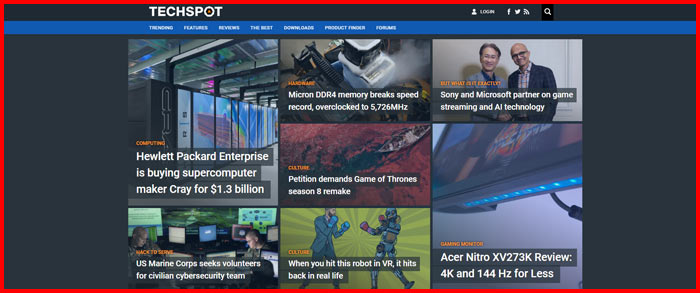This detailed caption provides an in-depth description of the image as follows:

The image is from the Techspot website. Encased in a red border, the layout is organized and sleek. At the very top of the image, there is a horizontal black bar featuring the website's name, "Techspot," displayed in white text with a small red accent in the "O." The interface includes options to log in, a prominently placed search bar, and a menu with various categories such as "Features" and "Reviews."

Within the central content area, which has a black background, multiple images and headlines are displayed. The first headline reads, "Hewlett Packard Enterprises acquires supercomputer maker Cray for $1.3 billion," and the subsequent line mentions, "U.S. Marine Corps seeks volunteers for a civilian cybersecurity team." Above these, another headline states, "Micron memory breaks speed record." Another notable headline reads, "Petition demands Game of Thrones remake," followed by an intriguing note, "When you hit this robot in VR, it hits back in real life," accompanied by a computerized image showing two robots engaged in a fight.

On the right side of the image, a headline announces, "Sony and Microsoft partner on game streaming and AI technology," accompanied by a photo of two men. Lastly, the final box features a review of the Acer Nitro, described with "144Hz display for less."

This comprehensive representation covers the website's branding, navigation, and highlighted news and reviews.